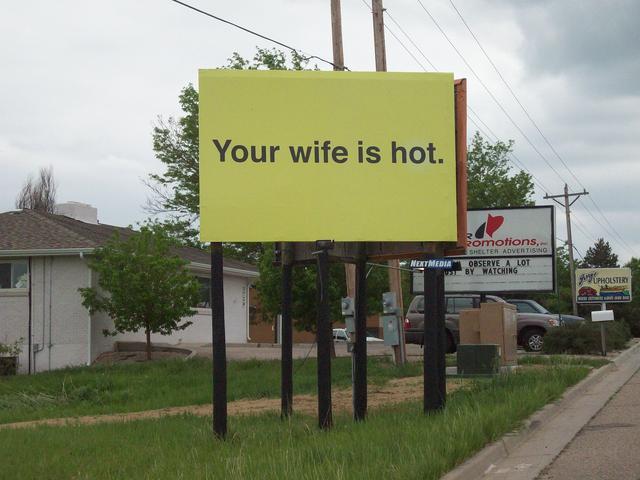The image is a close-up of a very small yellow billboard on the side of a concrete-paved road, supported by black wooden stilts. The billboard prominently displays the black text, "Your wife is hot." Below this main billboard, a small light is centrally positioned. Adjacent to this sign, another billboard is visible at an angle, forming a V-shape where the bottom tip points to the left. To the right of the scene, part of a street is visible, along with power lines running parallel to it.

In the background, another small business sign carrying the text, "You observe a lot just by watching," is displayed in plastic letters on a letter board. Behind this, a distant sign advertises an upholstery shop. On the left side of the image, there is a small white one-story building, possibly a house or a store, with a tree and at least one brown station wagon parked in front. Power poles and lines are scattered throughout the background of this daytime, possibly cloudy scene.